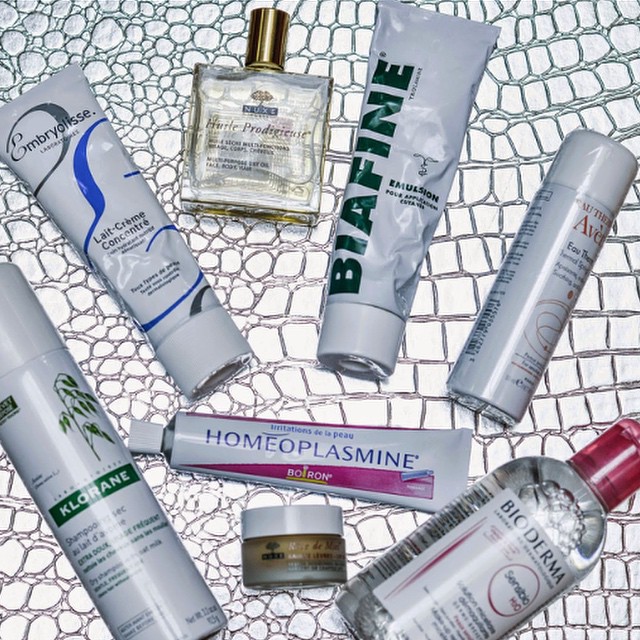This is a detailed downward shot of an array of cosmetic items strategically placed on a silver surface adorned with an alligator pattern, accentuated by black or different shades of silver. The assortment comprises lotions and spray products, including spray bottles, tubes, and a pump bottle located at the bottom right. Centrally positioned at the bottom, there is a jar with a white cap containing a tan substance, presumably foundation.

From left to right, forming a circular arrangement, the items include:
1. A white spray can with green printing.
2. A white tube featuring blue and gray designs and printing.
3. A clear bottle capped with gold.
4. Another white tube, this one with dark green printing.
5. A white spray can with black and red printing.
6. On the far right, a clear bottle filled with a clear liquid and capped with pink.

Horizontally aligned with the foundation jar is a plastic or metal tube decorated with white printing on a pink design. The combination of detailed packaging and the textured, exotic backdrop encapsulates a sense of elegance and functionality within the realm of skincare and beauty.